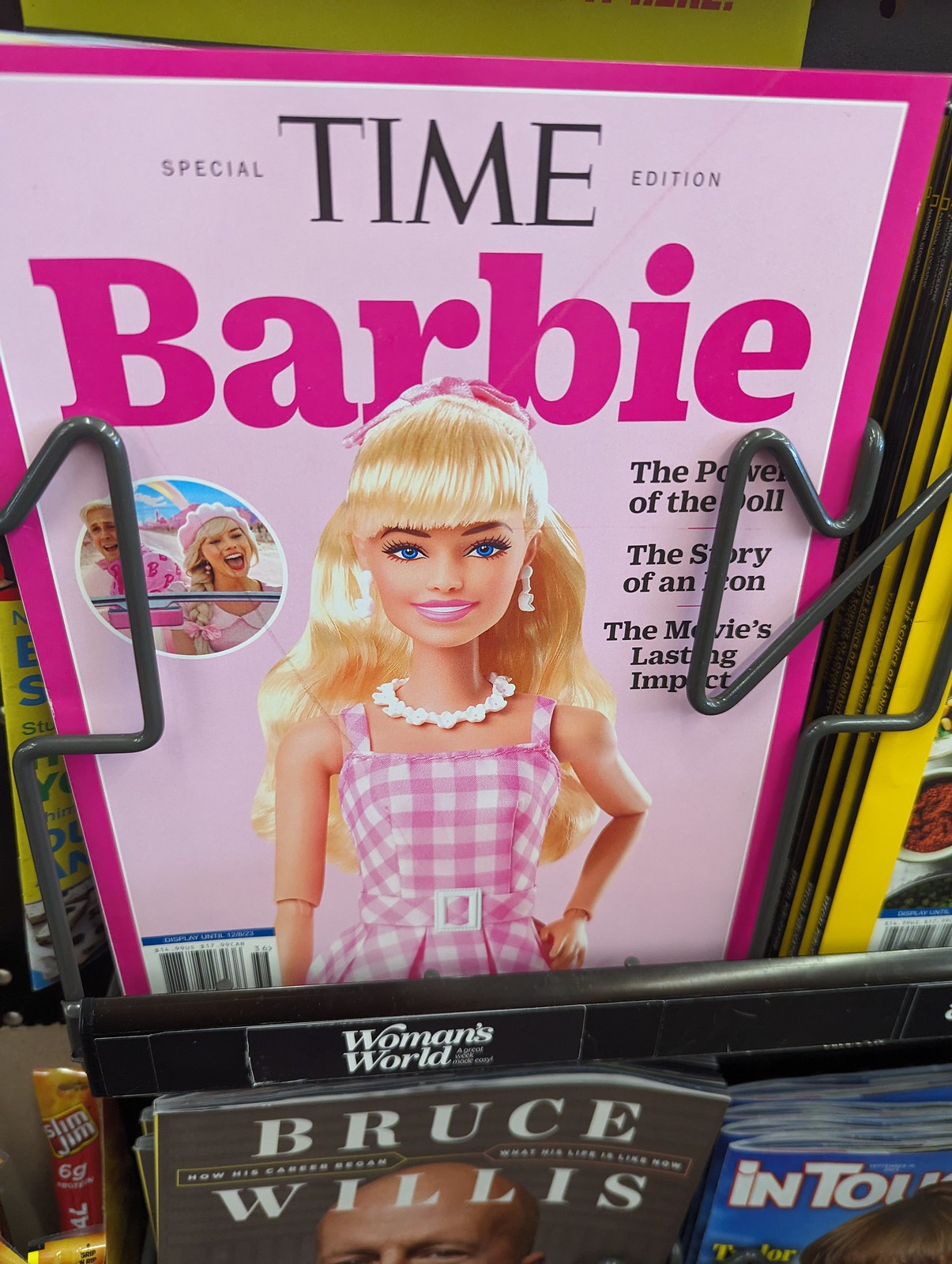This image showcases a magazine rack prominently featuring a special Time magazine edition dedicated to Barbie. The cover is predominantly pink with a lighter pastel shade filling the center and a darker pink border. The text at the top reads "Special Time Edition" with "Barbie" written in a matching pink hue just below the Time logo. Centered on the cover is a blonde Barbie doll dressed in a pink and white plaid dress, accessorized with a white necklace. She has blue eyes and pink lipstick. To her left, there is a small circular thumbnail of Ken and Barbie, likely depicting Margot Robbie and Ryan Gosling from the latest Barbie movie. The magazine cover is adorned with headlines on the right: "The Power of the Doll," "The Story of an Icon," and "The Movie's Lasting Impact." Below this Barbie-themed magazine, there is another magazine featuring Bruce Willis on the cover, distinguishable by its darker brown color. The rack itself is filled with additional magazines, emphasizing the Barbie special edition as the focal point.